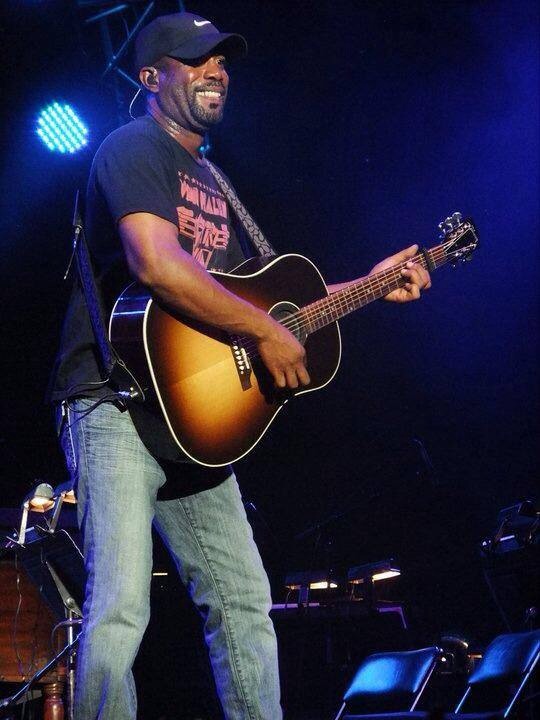In this image, an African-American man, who bears a resemblance to a younger Darius Rucker, is on stage playing an acoustic guitar. He wears light blue jeans, a black t-shirt with pinkish-red writing that is hard to read, and a black cap with a white Nike logo. His guitar features a dark brown top and edges, with a lighter yellowish-brown area just below the strings, and is held by a black and gray strap. He strums the guitar with his right hand while holding the notes with his left. The background is dark, but a series of blue lights and a spotlight are visible on the left side. There are musical instrument gear behind him and black folding chairs in the bottom right corner. He has a mustache and goatee, and the guitar appears to be plugged into an amplifier, suggesting he might be in a recording studio or performing on stage with friends, though no microphone is noted.